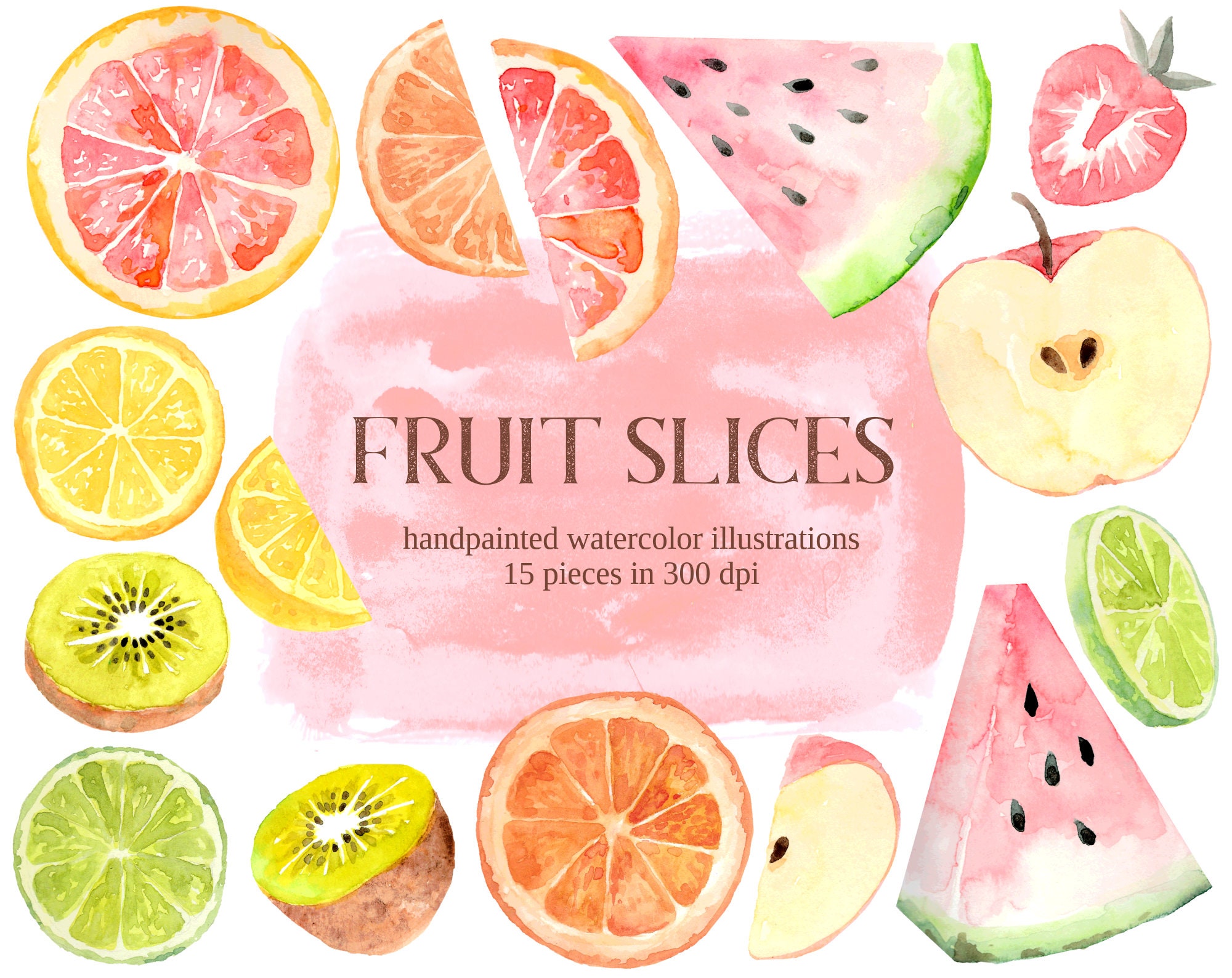The image appears to be a cover page for a book or similar product, featuring hand-painted watercolor illustrations of various fruit slices. A pink, amorphous rectangular watercolor background is centrally located, overlaid with text that reads "Fruit Slices," "hand-painted watercolor illustrations," and "15 pieces in 300 DPI." Surrounding this central text are detailed illustrations of fruit slices arranged in a clockwise fashion. Starting from the top left, there is a grapefruit slice, followed by a halved orange slice, another halved grapefruit slice, a watermelon slice, and a strawberry. Moving down the right side, the sequence continues with a halved apple, a lemon slice, and another watermelon slice. Along the bottom, there are slices of an apple, an orange, a halved kiwi, and a lime. Finally, going up the left side, the arrangement includes another kiwi slice and several lemon slices. The collectively vibrant and detailed watercolor art of grapefruit, lemons, kiwis, oranges, limes, apples, strawberries, and watermelons creates an eye-catching border around the central text.